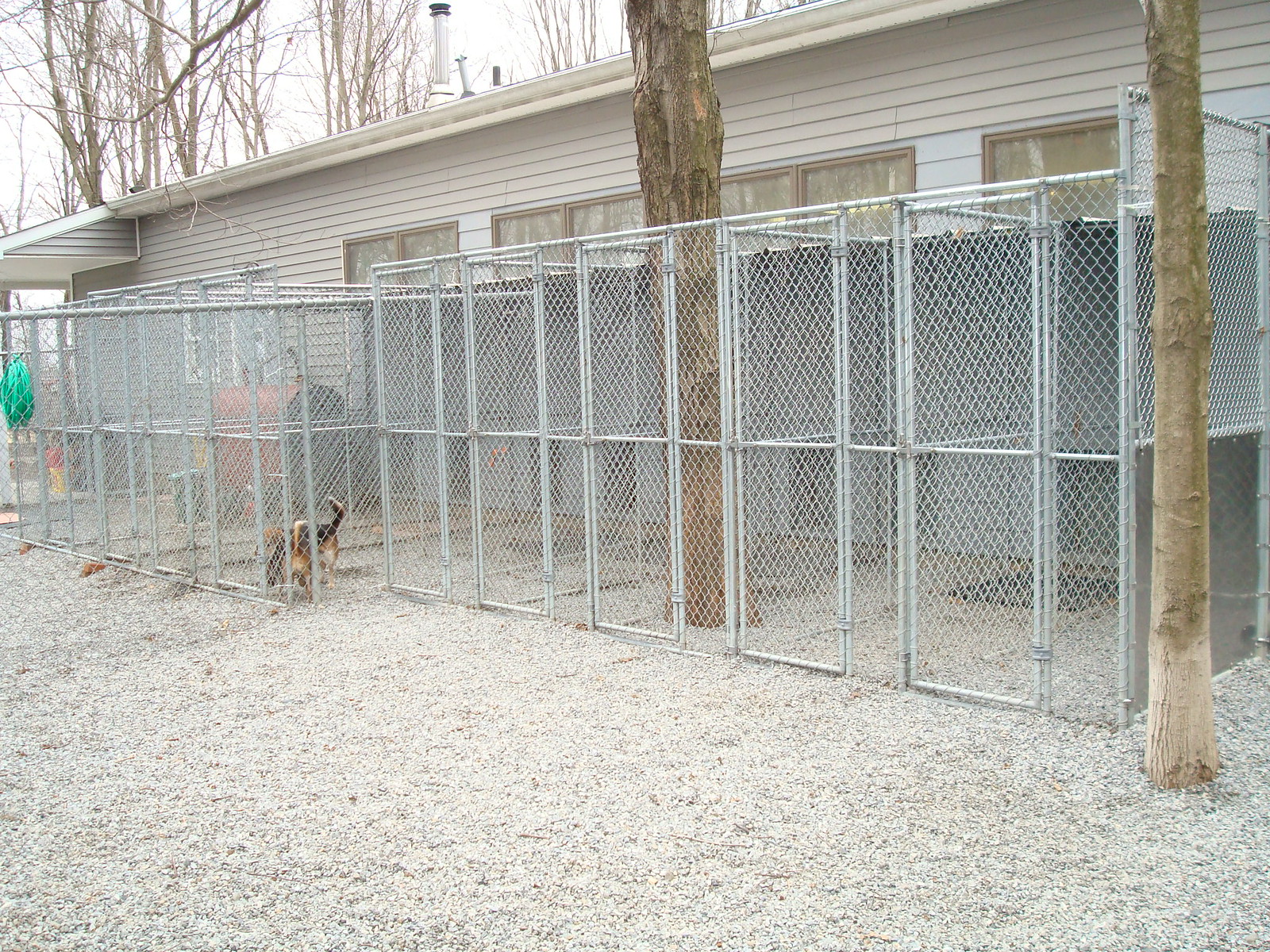This outdoor photo captures a row of metal wire mesh kennels lined up beside a white building, possibly a dog pound or animal rescue center. The ground is covered with small white pebbles that extend underneath the kennels. Each kennel has a doorway that might connect to indoor spaces, resembling windows or doggie doors. Cyclone fences structure the kennels, and a green garden hose is neatly rolled up on the far left side of the image. Notably, one kennel houses a dog that appears to be either a Beagle or a Basset Hound, characterized by its pronounced tail with a white tip and floppy ears. Scattered throughout the scene are dead or dormant trees, indicating a winter setting. In particular, one tree is inside a kennel close to the building, while another is to the far right. The barren trees in the background further emphasize the wintry atmosphere.